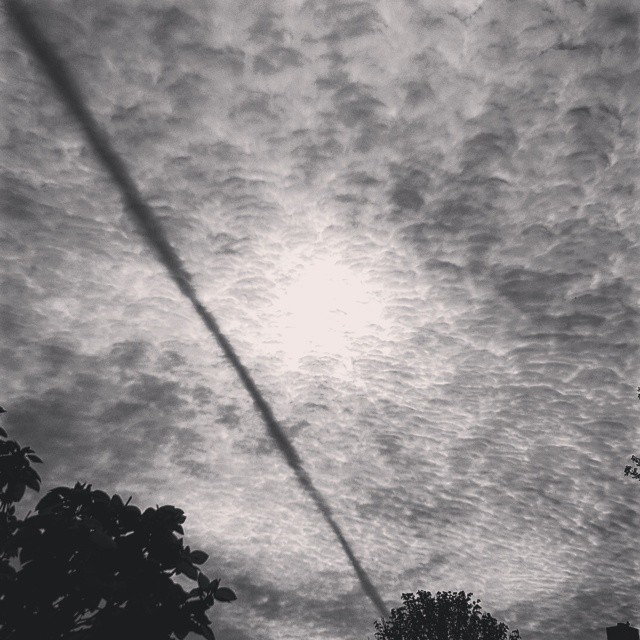This black and white photograph captures a dramatic sky scene. At the bottom of the image, a line of trees frames the composition, their silhouettes providing a stark contrast against the sky. Dark clouds dominate the upper portion, through which a bright, almost blinding light—most likely the sun—pierces the gloom, creating a striking focal point. A long line, possibly a telephone wire, stretches across the image, adding a linear element that guides the eye. Shadows of trees and a pole are subtly visible, enhancing the depth and complexity of the scene.